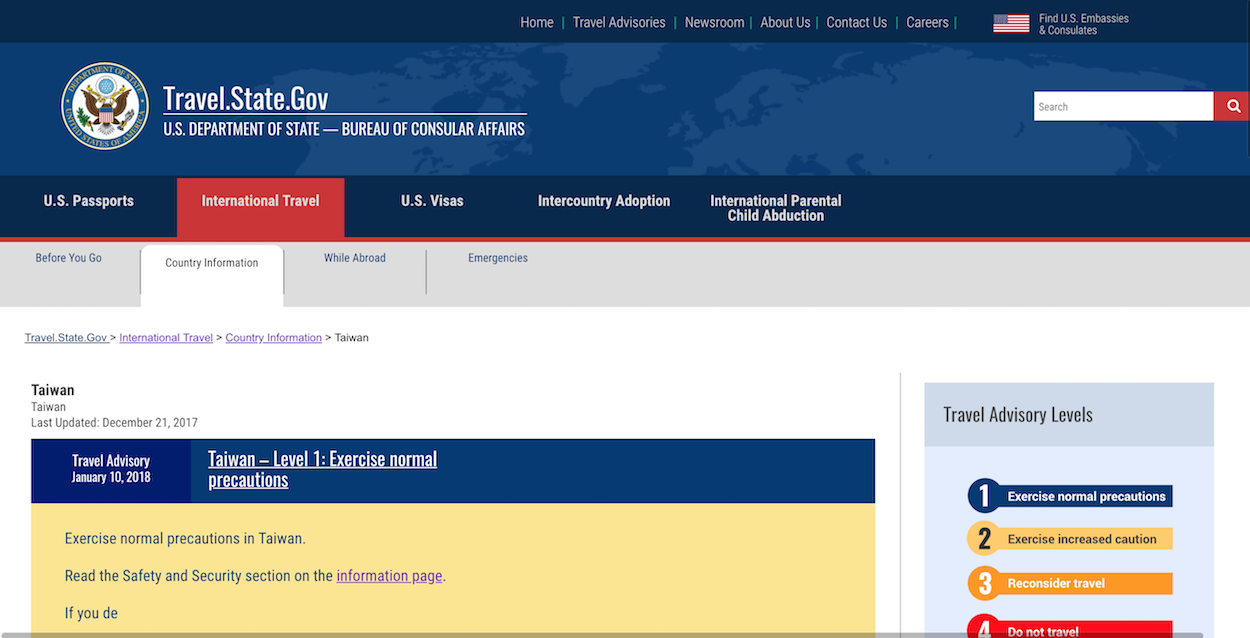The image captures a detailed view of the official website for the U.S. Department of State - Bureau of Consular Affairs. In the upper left corner, there is the Department's seal, featuring the emblematic eagle. Adjacent to the seal, the website heading reads "travel.state.gov." Below this heading, a dark blue navigation banner spans across the page, displaying various sections titled: U.S. Passports, International Travel, U.S. Visas, Intercountry Adoption, and International Parental Child Abduction. Notably, the "International Travel" tab is highlighted in red, indicating it is the currently selected section.

Beneath this, the page features a travel advisory dated January 10, 2018, for Taiwan, labeled as "Level 1: Exercise Normal Precautions." This advisory is prominently displayed to inform travelers about the safety status of their destinations.

On the lower right side of the webpage, there is a box titled "Travel Advisory Levels," outlining the four possible advisory levels. The levels are color-coded for easy identification: 
1. Level 1: Exercise Normal Precautions (dark blue background)
2. Level 2: Exercise Increased Caution (bright yellow background)
3. Level 3: Reconsider Travel (orange background)
4. Level 4: Do Not Travel (red background)

This webpage is a key resource for travelers seeking up-to-date advisories and safety information for international travel.